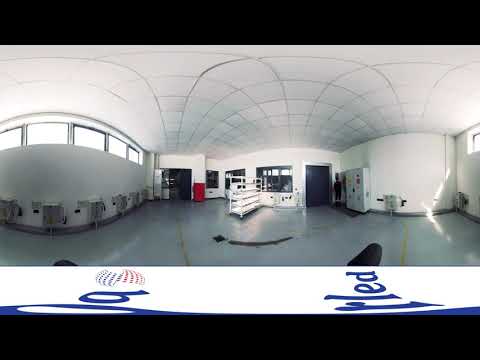The image depicts a spacious, plain room with white walls and a tiled ceiling, resembling a basement storage area or locker room. The floor is white with noticeable yellow stripes. The left side features a row of six gray sinks and a partially visible open black door, next to which sits a red cabinet or drawer. Adjacent to this area, a blue door and three reflective windows line the wall, accompanied by white shelving units. On the far right side of the room, a long wall with windows at the top is observed, along with another black door next to a mysterious red barrel. The room's cement floor and overall minimalist design suggest it might serve a practical, utilitarian purpose.